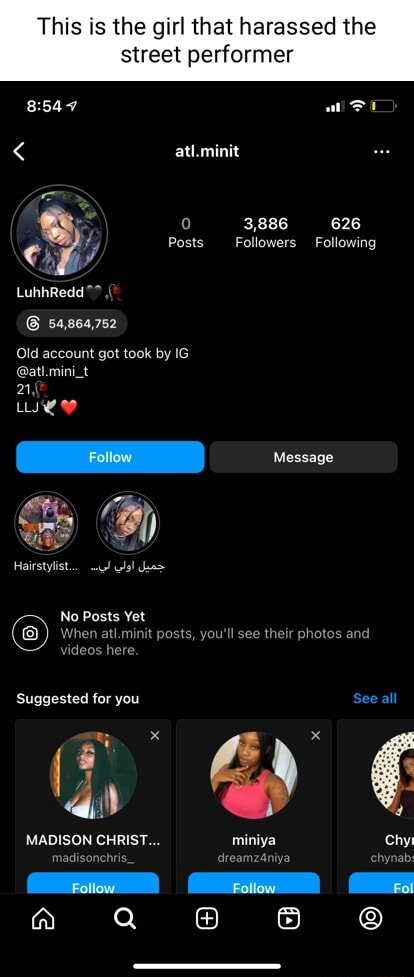The image captures a close-up shot of a smartphone screen against a completely black background. The time displayed at the top of the screen is 8:54, and the battery indicator, highlighted in yellow, signals that the battery is nearly depleted.

Prominently featured at the top portion of the screen is a profile picture of a woman. Above her image, the username "Loon Red" is displayed, possibly indicating her name or a nickname. Detailed account statistics are visible, showing zero posts, 3,886 followers, and 626 accounts she is following.

Above the smartphone screen, in black text, there's a statement mentioning, "This is the girl that harassed the street performer." Further down on the screen, a comment notes, "Old account got took by IG," suggesting her previous account was deactivated by Instagram. Additional information includes "Admin 21" accompanied by a heart emoji. 

At the bottom of the screen, the account status indicates "No posts yet," and there is a section labeled "Suggestions for you" offering recommendations for other profiles to follow.